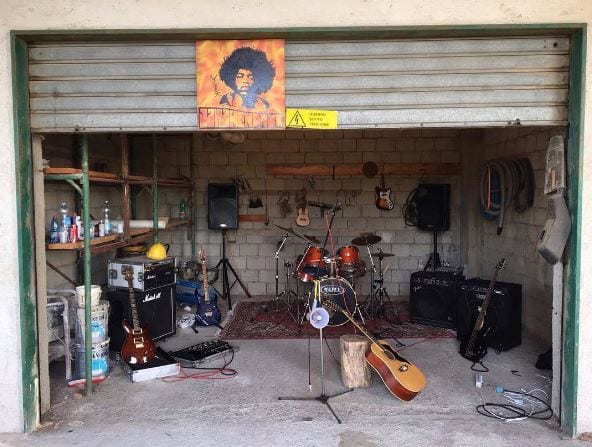This image depicts a garage repurposed as a band rehearsal space. The garage door, made of slightly rusted silver metal, is open about three-quarters of the way. Near the top of the door, slightly left of center, hangs a Jimi Hendrix poster with a black silhouette of the musician against an orangey-red tie-dyed background, and text that reads "Jimi Hendrix." To the right of the poster is a small yellow sign featuring an electrical hazard symbol. 

Inside the garage, the concrete floor and grey brick walls frame an array of musical equipment. On the left, scaffolding supports two shelves, the upper one mostly empty, while the lower shelf holds assorted bottles and some paint tins below. A Marshall guitar amplifier with a brown Paul Reed Smith guitar leaning against it is also positioned on this side, accompanied by a large pedal board on the floor.

At the back of the garage, two PA speakers on stands flank the space, with three horizontal wooden planks against the wall suspending more instruments. A ukulele is mounted on the middle plank, while the upper plank holds what appears to be a small plastic electric guitar, possibly from the Guitar Hero game. A brown five-piece Tama drum kit, complete with cymbals, occupies the center back, and to the right of it stands a Fender amplifier. Further right, near the garage's front corner, sits another amplifier, likely a Peavey, with a black bass guitar in front. 

In the center of the garage, a microphone on a stand takes prominence, featuring a hanging megaphone and a cord. Nearby, a tree stump possibly used as a seat supports a leaning twelve-string acoustic guitar. The setup, complete with various cables and power boards scattered on the floor, clearly indicates this garage serves as a well-equipped rehearsal space ready for a band to practice.